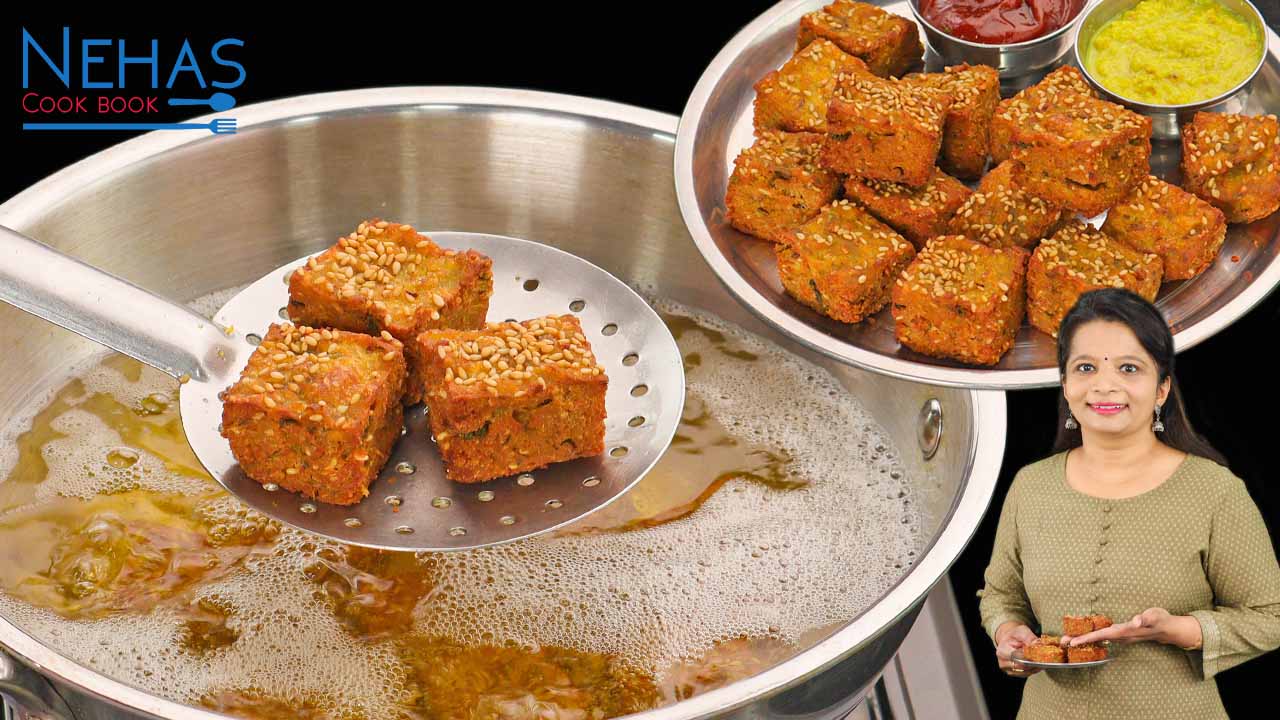The image depicts two large stainless steel pans, filled with bubbling oil and frying cubes of tofu, covered in sesame seeds. In the forefront, a slotted stainless steel spatula drips oil as it lifts a batch of crisp tofu pieces. Beside the pans sits a silver plate, neatly arranged with the tofu squares and accompanied by two sauces in small containers—one red, one yellow. In the bottom right corner stands a woman, likely Neha, holding a plate of the sesame tofu, smiling as if explaining the dish. The top left corner of the image features the title "Neha's Cookbook" in blue and red fonts, embellished with graphics of a spoon and a long fork. The background is a stark black, making the vibrant details and sizzling food the focal points of this enticing scene.